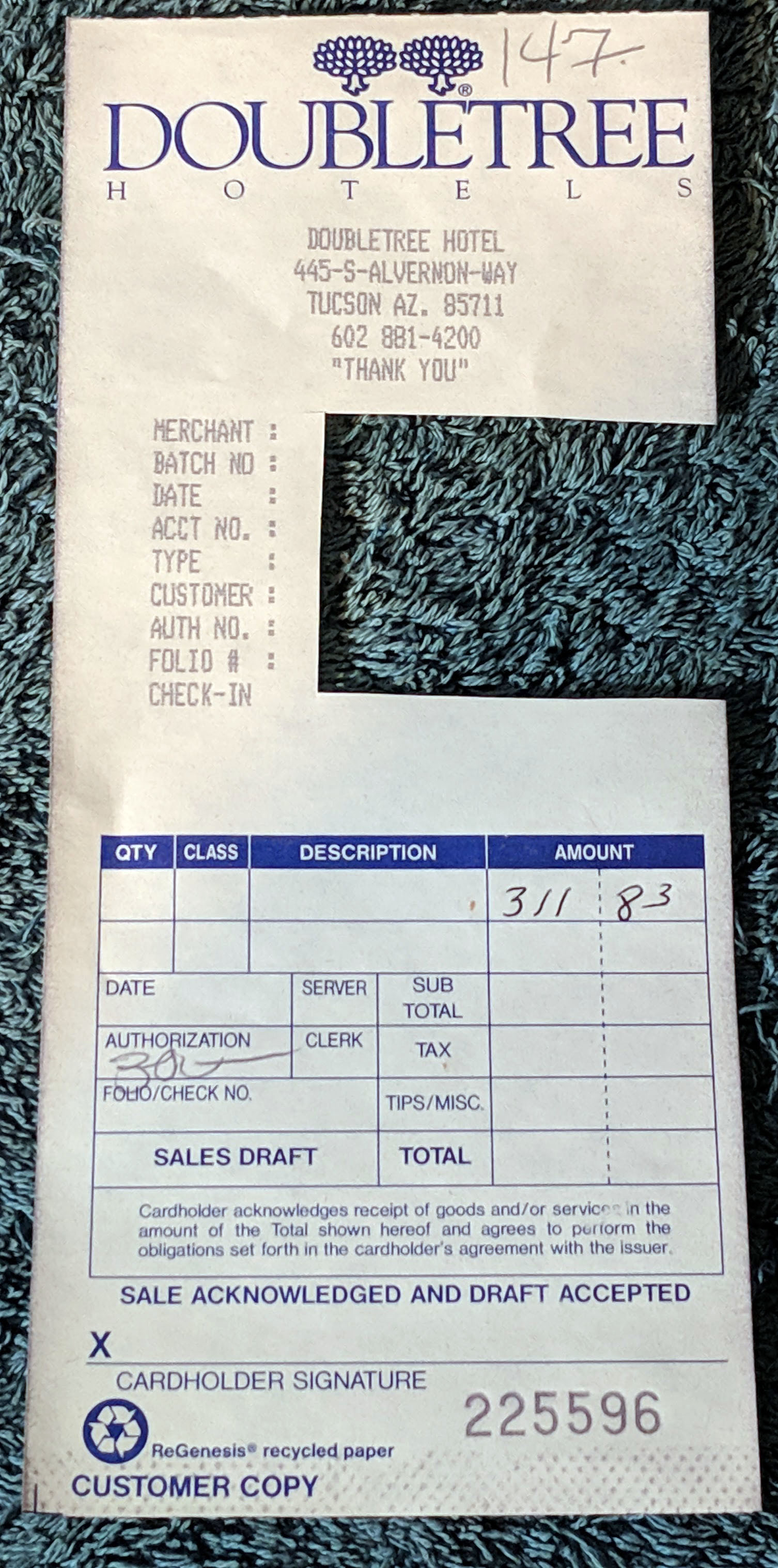**Caption:**

A close-up shot of a receipt lying on a blue shag rug. The top of the receipt prominently features the blue logo and text of Doubletree Hotels. Above the "Doubletree" text, two chandeliers and the number "147" are handwritten in pen. Below the logo, the hotel's address is clearly printed: "Doubletree Hotel, 445 S Alvernon Way, Tucson, Arizona 85711," followed by the phone number "602-881-4200" and a courteous "Thank you" enclosed in parentheses.

On the left side of the receipt, categories such as merchant, merchant batch number, date, account number, type, customer, auth number, folio number, and check-in are listed sequentially, although no data is present next to these headings—indicating that part of the receipt has been cut off. Further down, there is an outlined section detailing the charges and a designated space for the cardholder's signature.